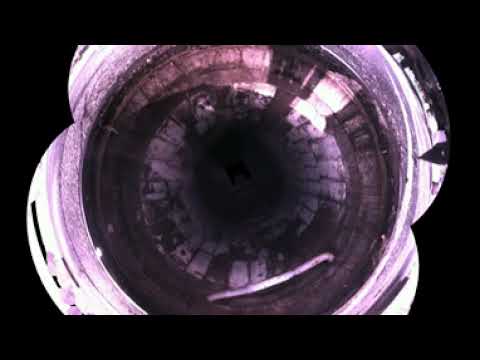The image features a central object resembling a stylized flower or donut, positioned within a black rectangular background. The background is divided into three vertical panels: a dominant central black panel flanked by narrower, slightly lighter black or gray panels. The centerpiece of the image is a light purple and gray flower-like object with four petal-like bevels. The object is made of a hard material, possibly concrete or plaster. At its core is a circular area with a dark, pupil-like inner circle surrounded by a light purple outer ring that contains small white rectangles of light, giving it a luminous appearance. The object stands out starkly against the dark backdrop, devoid of any text, writing, or people.